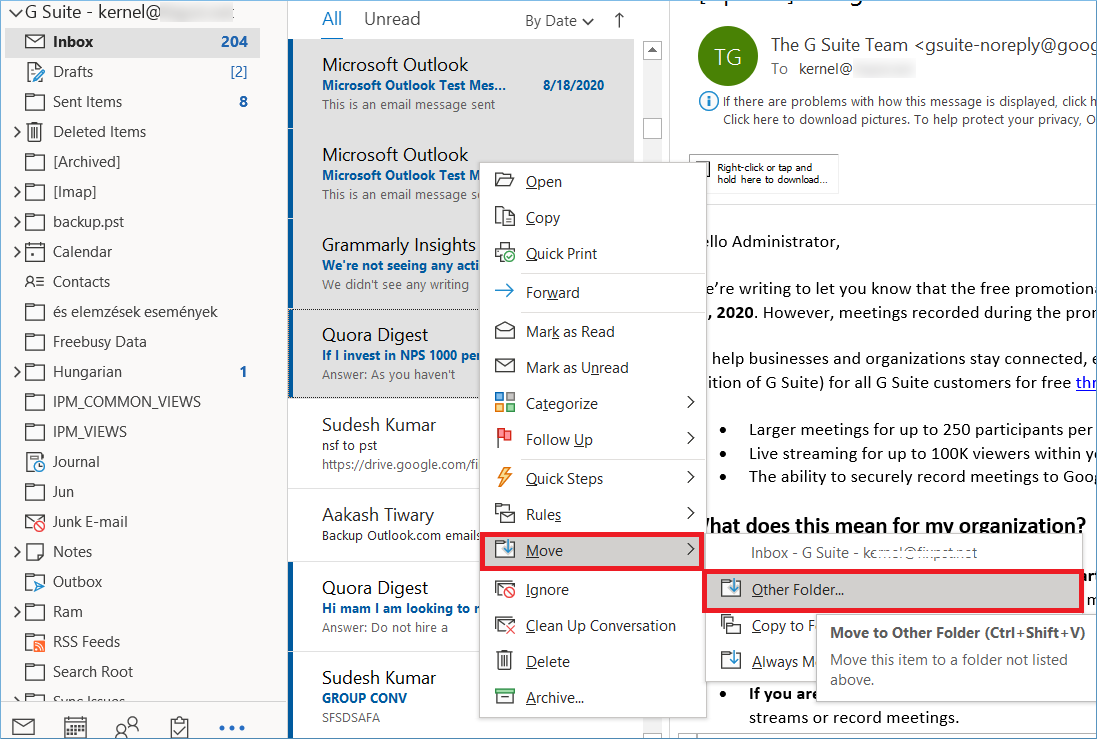The image features a white background and is approximately 20-30% wider than it is tall. It is segmented into three sections: left, center, and right. The left section occupies roughly 30% of the width, while the center and right sections each take up about 35%.

The content displayed appears to be a screenshot of an email program, possibly a rudimentary version of Gmail. In the upper left corner, there is plain black text with a down arrow, followed by "G Suite-Kernel" and a grayed-out email address, suggesting this is a G Suite interface.

The left column serves as a navigation menu featuring a list of typical email folders and other navigation items. These include:

- Inbox
- Drafts
- Sent Items
- Deleted Items
- Archived
- IMAP
- Backup.pst
- Calendar
- Contacts
- An item in another language
- Free Busy Data
- Hungarian
- IPM Common Views
- IPM Reviews
- Journal
- JUN
- Chunk Email
- Notes
- Outbooks
- RAM
- RSS Feeds
- Search Root

Each of these items is accompanied by icons to their left. The interface is predominantly in black and gray, with minimal use of color, distinguishing it from the more visually dynamic, traditional web-based Gmail layout. Not all menu items are fully readable, as some extend beyond the visible area.